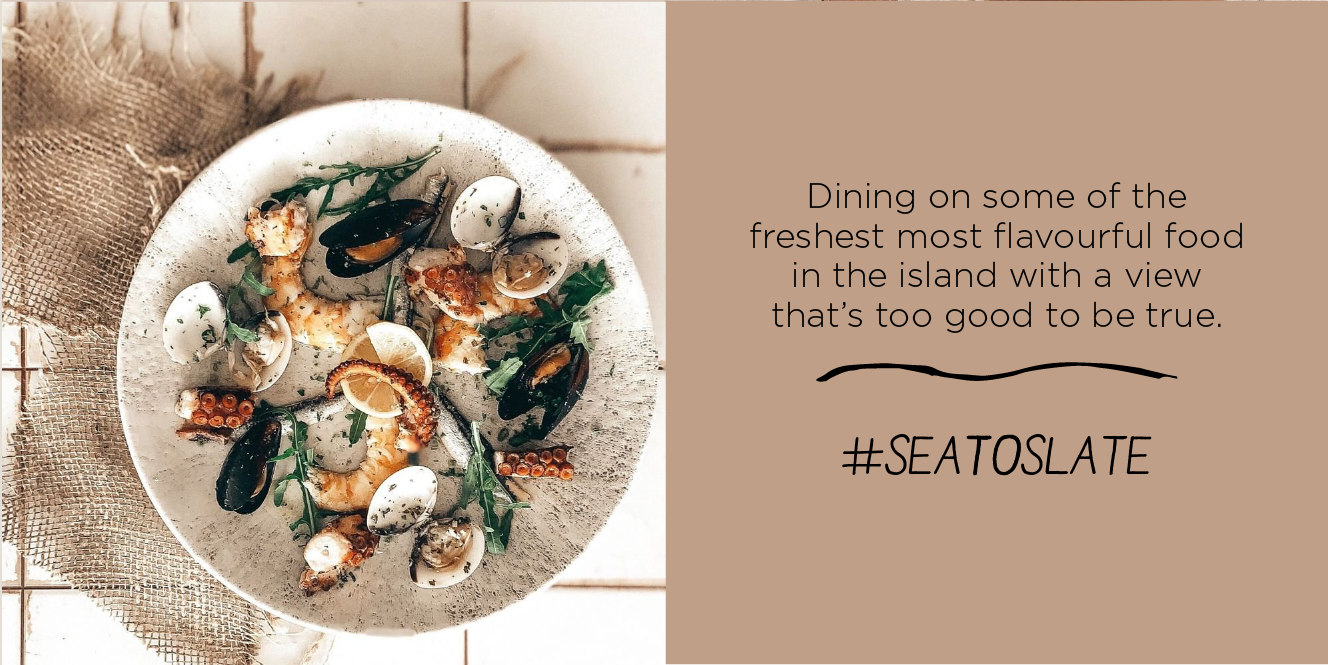A rustic seafood feast is elegantly laid out on a white square tile countertop, showcasing a picture of someone's dinner in the advertisement header image. Despite the slightly worn and messy grout lines between the tiles, the scene exudes a charming, lived-in feeling. A piece of burlap, possibly a ribbon, is casually tucked under a weathered stoneware plate, adding to the rustic aesthetic. The plate is adorned with succulent seafood, including squid tentacles, clams, oysters, and fresh herbs, all accented with vibrant slices of lemon. To the right, on a tan background that perfectly complements the burlap, a caption reads: "Dining on some of the freshest, most flavorful food on the island with a view that's too good to be true." A delicate squiggle line separates this text from the campaign hashtag, #SeatoSlate.